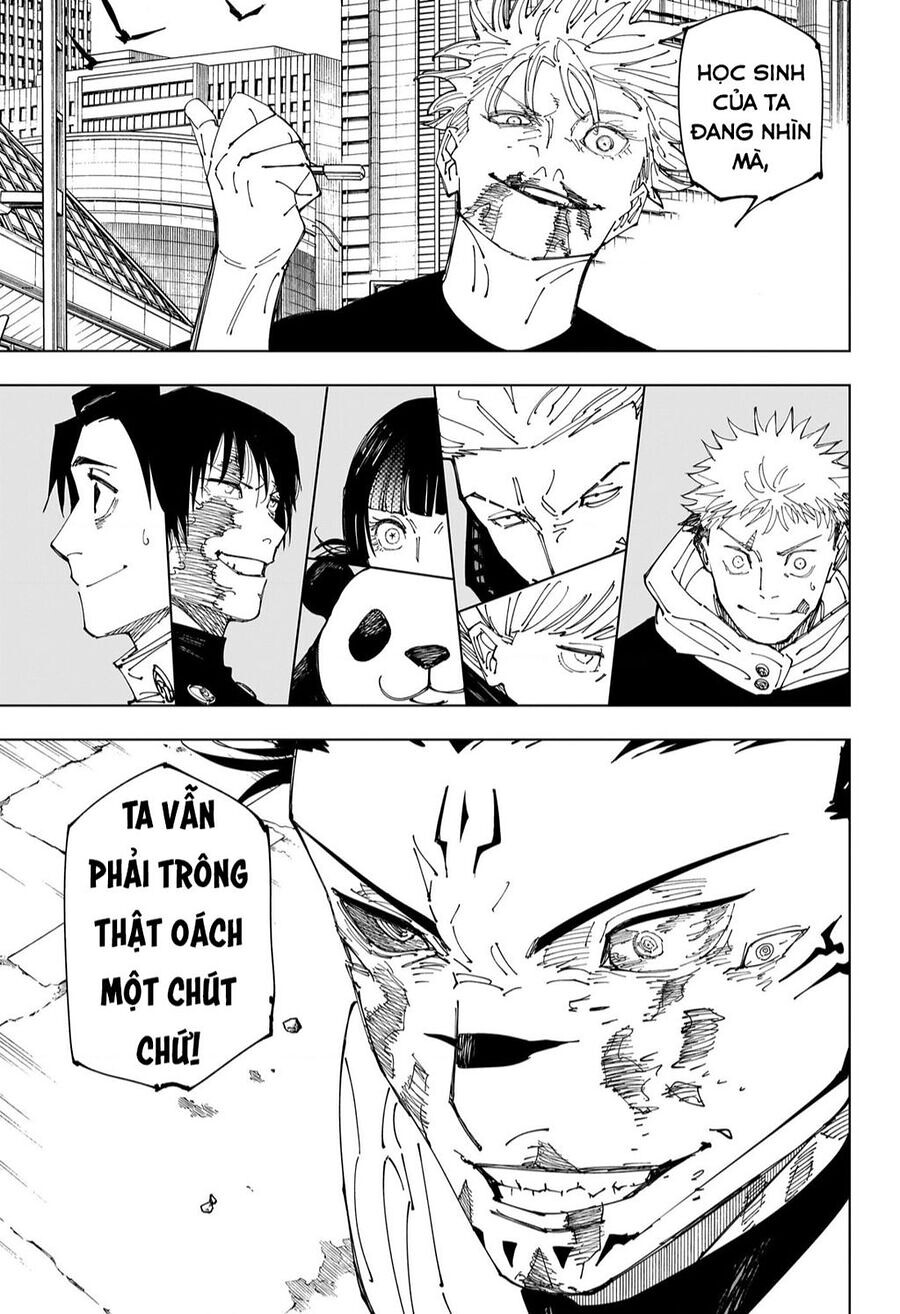This black and white manga page is divided into three distinct panels. In the top panel, there is a young man with short hair and unusual bird-like marks around his chin and mouth. He stands in front of a city skyline visible through a window and points his thumb backward, with a speech bubble in Vietnamese that reads, "Hoc Sinh Qua Tha Thanh Ninh Ma." The middle panel consists of seven smaller sub-panels showcasing various hand-drawn faces and reactions, including a panda. These reactions appear to be directed towards what the young man in the first panel has said. The bottom panel provides a close-up of a menacing figure with three eyes, a cut on his nose, and burns across his cheeks, mouth, and eyes. Additionally, there are marks on his forehead and next to his ear, with another speech bubble in Vietnamese that says, "Ta Van Phi Truong That Och Ma Choo Choo."